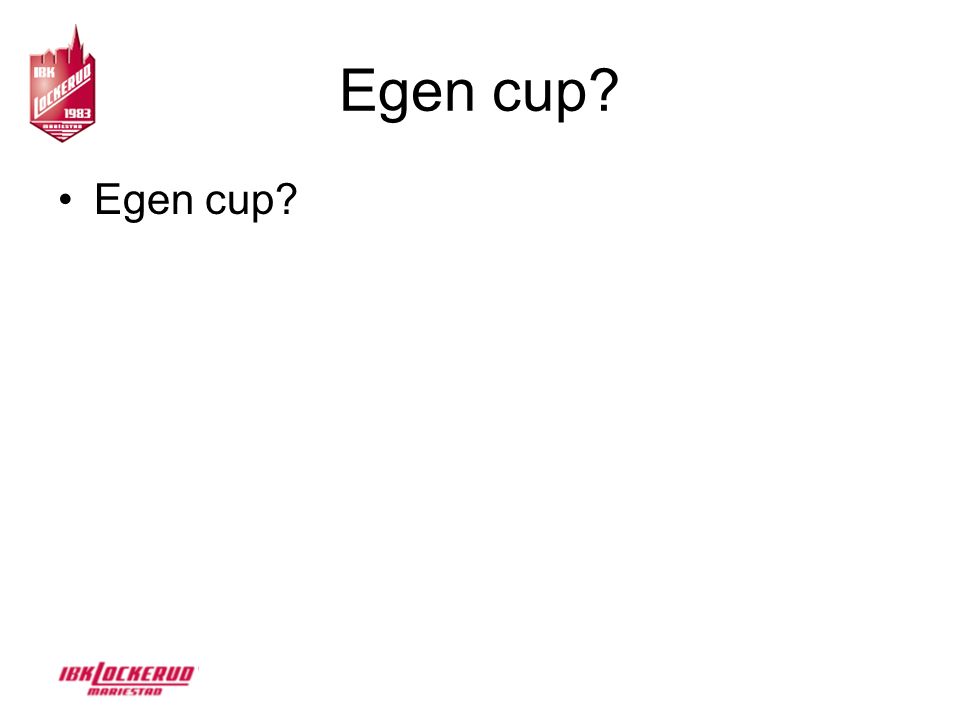The image appears to be an incomplete PowerPoint slide featuring minimal text and a logo. Centered at the top is the title "E-GEN-CUP" or "EGAN-CUP" followed by a question mark, which is repeated as the only bullet point on the slide, suggesting uncertainty about the term. The visual design is sparse, with a predominantly white or translucent background. In the upper left corner, there is a red emblem with white lettering depicting a town skyline, including a church steeple, representing a coat of arms or logo. The red emblem contains the text "I-B-K" followed by "LOCKERUO" and the year "1983." A similar identifier, "I-B-K Lockeruod Mari Stodd," appears in the lower left corner in plain red text. The overall impression is of a work-in-progress presentation slide or placeholder image, possibly for a brand or event associated with the given emblems and text.